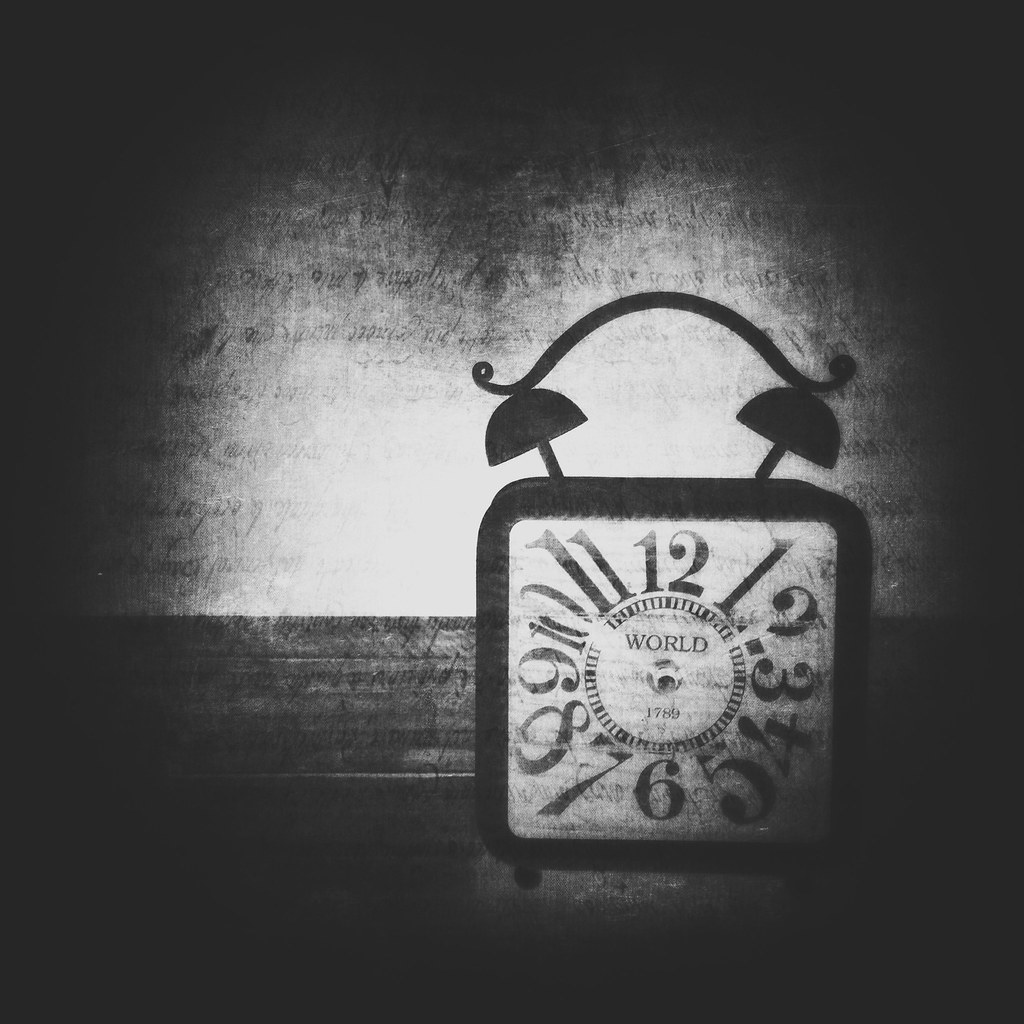The image, which appears to be a piece of digital art or a photograph, features an intricately designed, vintage-style alarm clock prominently positioned in a dimly lit room. The clock has a square face bordered in black, with a contrasting white background displaying numbers from 1 to 12. Notably, the numbers 1, 7, and 11 are significantly larger than the others. The center of the clock face contains the word "WORLD" in capital letters, along with the year "1789." A distinctive feature of the clock is its classic alarm bells connected by a swirly arcing black line and a V-shaped handle at the top. The surrounding environment is shadowy, with black edges and a faintly illuminated background in shades of white, gray, and black. There are also ambiguous text elements on the walls, but they are not clearly legible. Overall, the image focuses solely on the clock, with no other objects or people present, creating a stark and evocative visual composition.